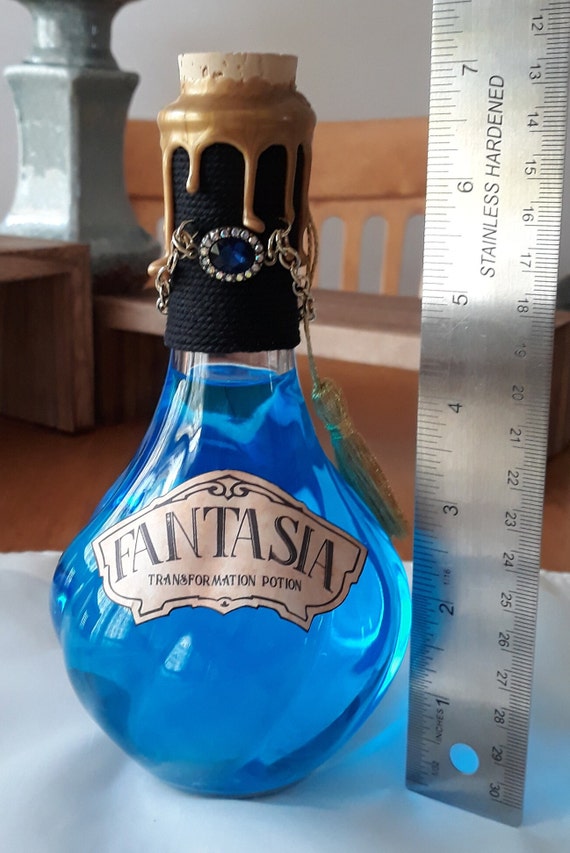This is a highly detailed color photograph featuring a clear glass bottle filled with a captivating turquoise-blue liquid. The bottle is sealed at the top with a cork, which is artistically adorned with golden wax dripping down its sides. Wrapped around the neck of the bottle is a black cord, elegantly accentuated by a central blue jewel encircled with sparkling rhinestones. From the right side of the neck, a metallic tassel dangles gracefully. The bottle bears a label that reads "Fantasia Transformation Potion." To the right of the bottle, a silver ruler stands upright, measuring the bottle's height at approximately 7 inches. Both the bottle and the ruler are placed on a pristine white surface, highlighting the intricate and enchanting details of the bottle.